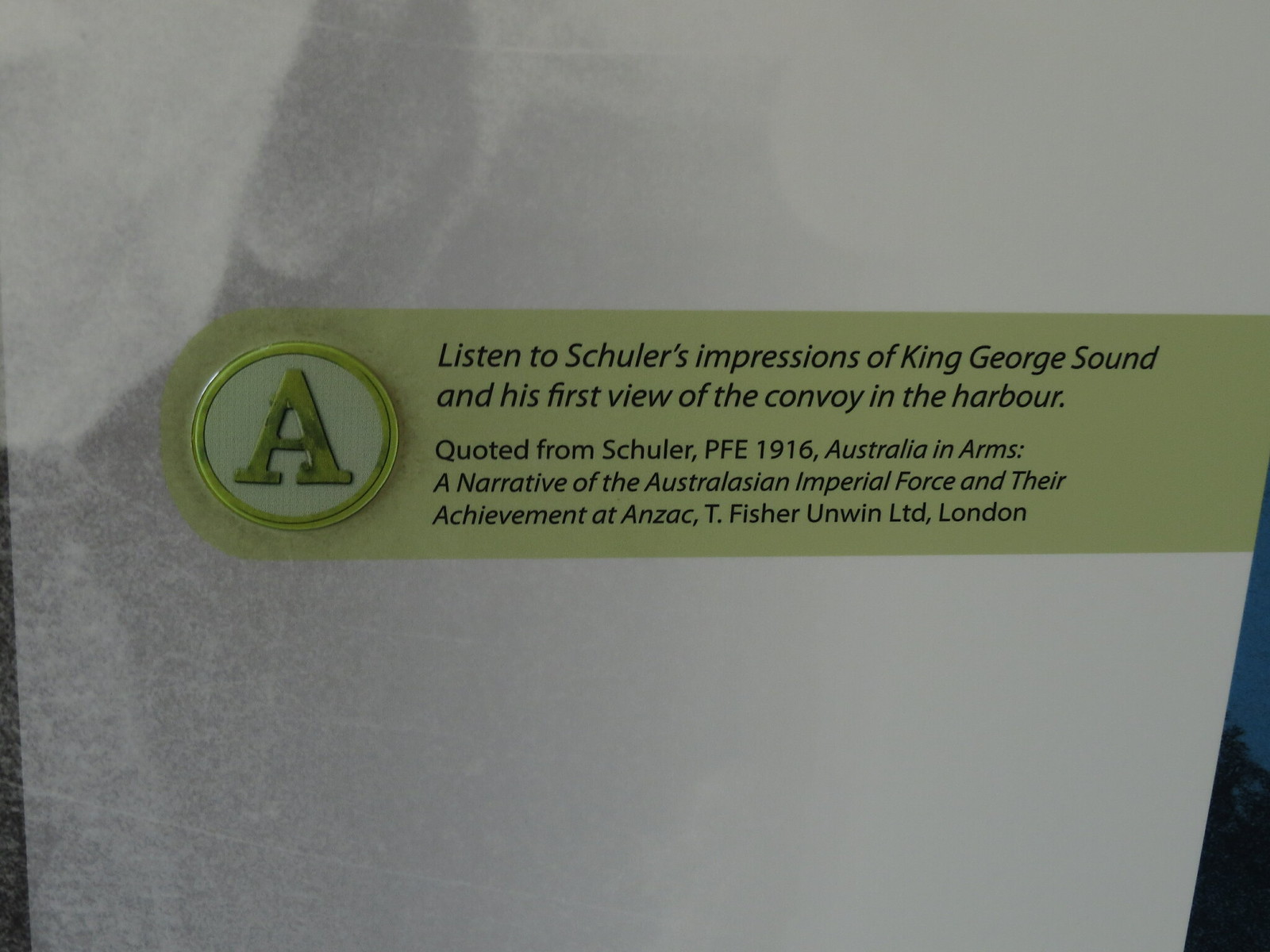The image features a white background with a textured appearance, reminiscent of marble or stone, and includes a subtle faded charcoal imprint that resembles a handprint. Spanning from the left to the right is a light green banner. On the left side of this banner is a circular area with a green border, containing a capital letter A in green, resembling the Times New Roman font, suggesting a physical button-like presence. To the right of this circle, within the green banner, is a block of black text that reads: "Listen to Schuller's impressions of King George Sound and his first view of the convoy in the harbor. Quoted from Schuller, PFE, 1916, Australia in Arms, a narrative of the Australasian Imperial Force and their achievement at Anzac, T. Fisher Unwin Limited, London."